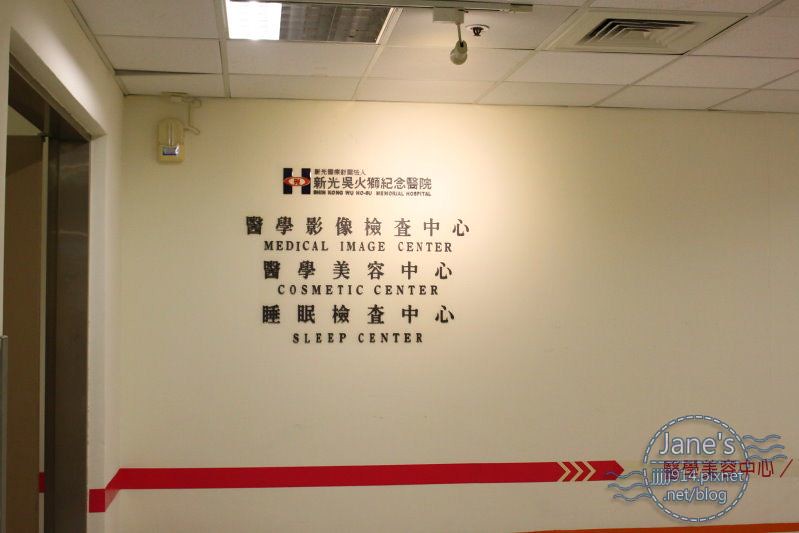A detailed caption for the image could be:

Inside a corridor of the Hong Kong Wu Wu Ho Boo Memorial Hospital, an institutional white wall displays important directional information in both Chinese and English. At the top, in small English font, is the text "Hong Kong Wu Wu Ho Boo Memorial Hospital" accompanied by Chinese characters and a small logo to the left. Below this, three lines of text provide the names of key facilities: "Medical Image Center," "Cosmetic Center," and "Sleep Center," each with their corresponding Chinese translations above them in larger fonts. A distinct red stripe, positioned about three feet off the ground, runs horizontally along the length of the wall and is accentuated by three small yellow arrows pointing to the right. These guide visitors towards a notable red-colored Asian text, with "James" and the partial URL "jjjj914.pixnet.net/blog" faintly visible beneath it. Adjacent to the left, there is a brown doorway, while the ceiling above is white and houses a spotlight casting light onto the text below.